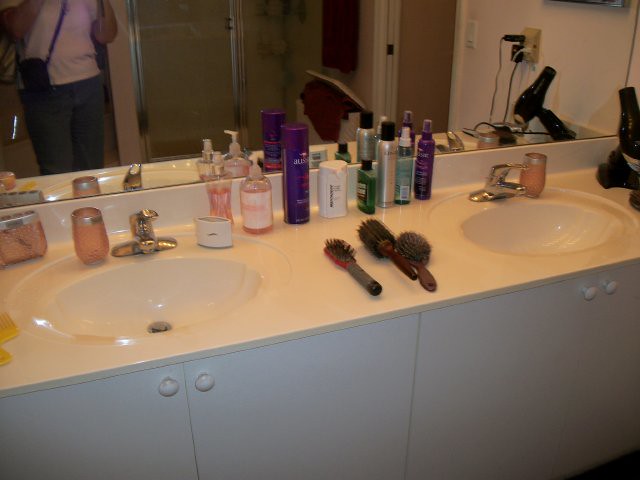This horizontal color photograph captures a dimly lit bathroom, highlighting its dual sinks, cabinetry, and mirror. The image quality is low due to insufficient lighting. In the background, a person with a white shirt, black pants, and a purse stands, taking the photo. Behind them, a partially visible shower features a glass enclosure framed with metal.

The focal point of the image is the dual sink setup, integrated seamlessly into a white countertop. Each sink is paired with single-handle, silver faucets that control hot, cold, and off functions. Below the sinks, wooden cabinetry boasts cabinet doors, each fitted with two knobs.

The countertop is cluttered with various items, including hairbrushes, soaps, and other toiletries. A hair dryer and another electrical device are plugged into an outlet on the wall. The bathroom walls appear white, complementing a white light switch and contrasting against a brown wooden door.